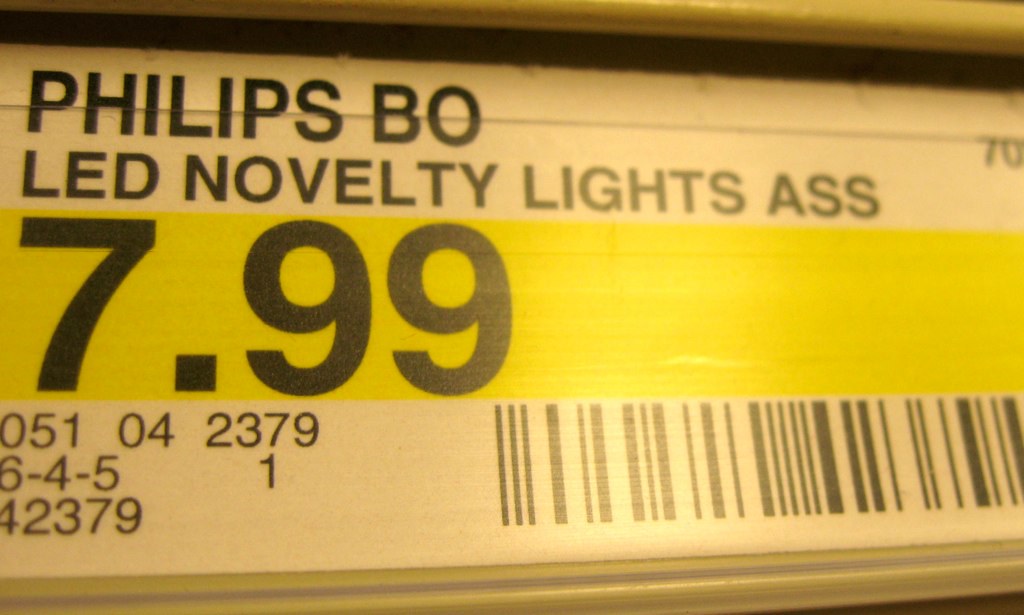This is a close-up photograph of a product price tag against a white background. At the top of the image, "Philips BO LED Novelty Lights ASS" is printed in black font. In the upper right corner, the number "70" is also displayed in black font. Below the Philips branding, a price label with a yellow background and black font prominently reads "$7.99". Underneath the price, there is a sequence of black numbers: "05104237964514237". On the left side of the image, part of a barcode is visible. The entire image includes a slight light glare, adding a reflective quality to the surface of the tag.